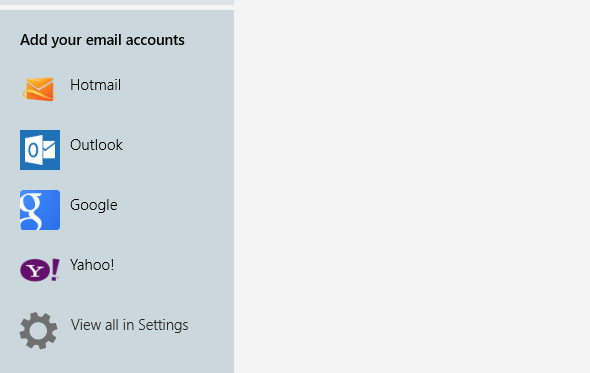The image displays a user interface for adding email accounts. On the right side of the image, occupying roughly 55-60% of the space, is a solid light grayish color. On the left side of the image, there is a vertically-oriented rectangular section. At the top left of this section, in black text, are the words "Add your email accounts."

Below this header, there are five distinct categories listed, each with corresponding icons:
1. **Hotmail**: Accompanied by an orange envelope icon, with the word "Hotmail" in black.
2. **Outlook**: Represented by a squared box icon containing a white envelope on a blue background, with the word "Outlook" in black.
3. **Google**: Denoted by a blue squared box icon with a white 'G' logo, and the word "Google" in black.
4. **Yahoo!**: Featuring the Yahoo! logo, a white 'Y' with an exclamation point, and the word "Yahoo!" in black.
5. **View all in settings**: Indicated by a gear icon next to the text.

The detailed arrangement and color scheme effectively guide users through the process of adding various email accounts.